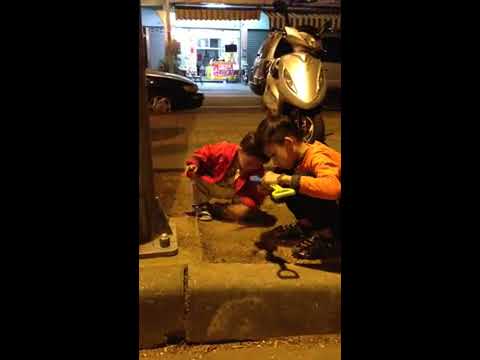This nighttime photograph captures two young children engrossed in play. They are squatting on a curb, with one child holding a neon green shovel with a yellow handle. The first child, positioned in the foreground, is a little boy with short dark hair, wearing an orange long-sleeved shirt, pants, and tennis shoes. He is looking down at the shovel in his left hand. Behind him is a slightly smaller child, also with short dark hair, wearing a red jacket and shorts, similarly focused on the shovel. The illuminated backdrop features a building with a red and white striped awning, partially obscured by the hood of a parked car. The scene is made even more intriguing by a gold item near the children and the faded, somewhat blurry quality of the image, suggesting an older photograph.